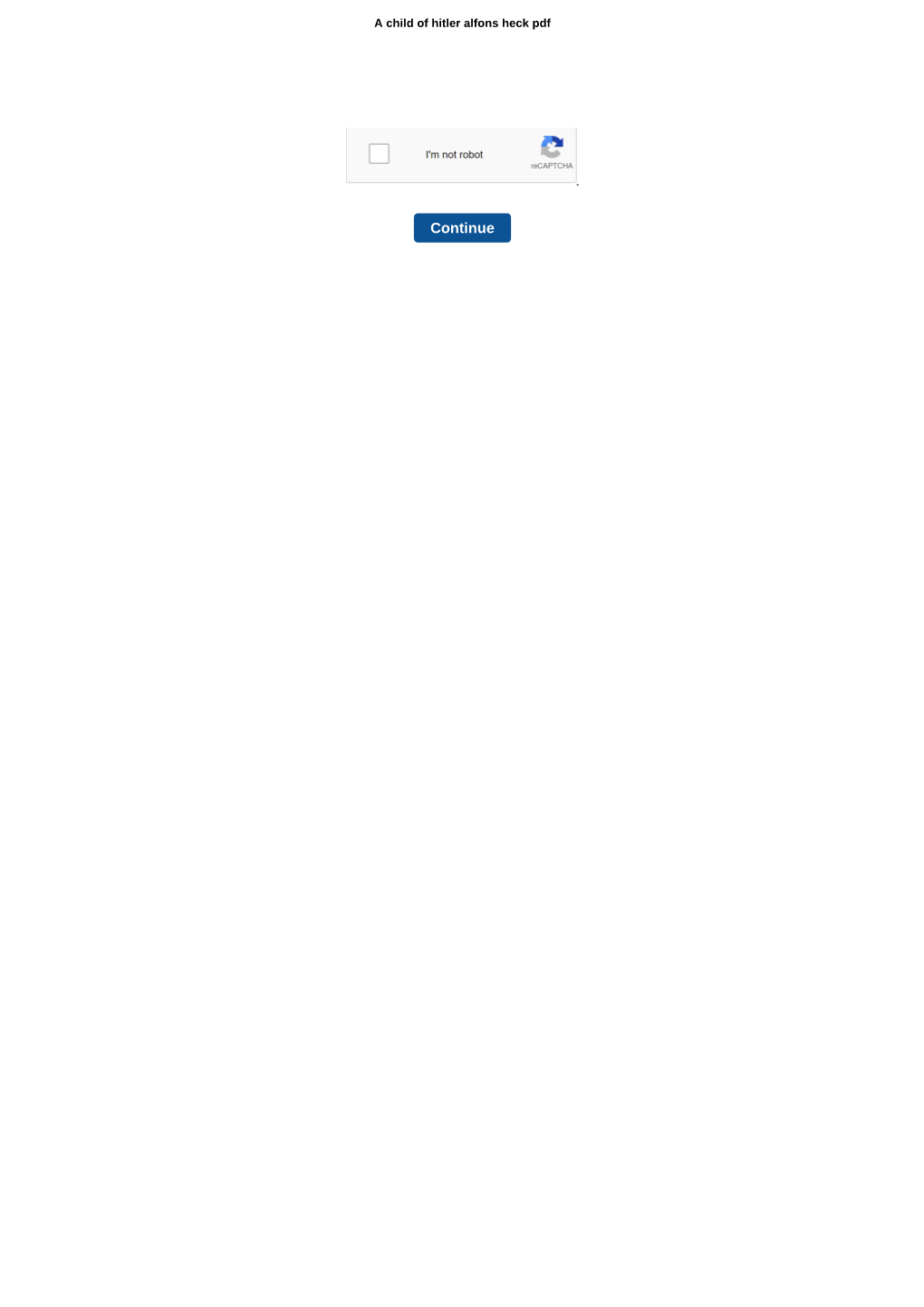In this image, we see a small print document displayed against a purple background. The text appears to reference "a child of Hitler at loss" and also mentions "pack pdf," though it is quite difficult to read due to the small and unclear print. Below the text, there is a purple box containing a CAPTCHA verification element, which includes a checkbox labeled "I'm not a robot" along with the CAPTCHA icon. Additionally, there is a prominent purple "Continue" button positioned beneath the verification box. The overall composition of the image is minimalistic and somewhat challenging to decipher due to the tiny and faint text.